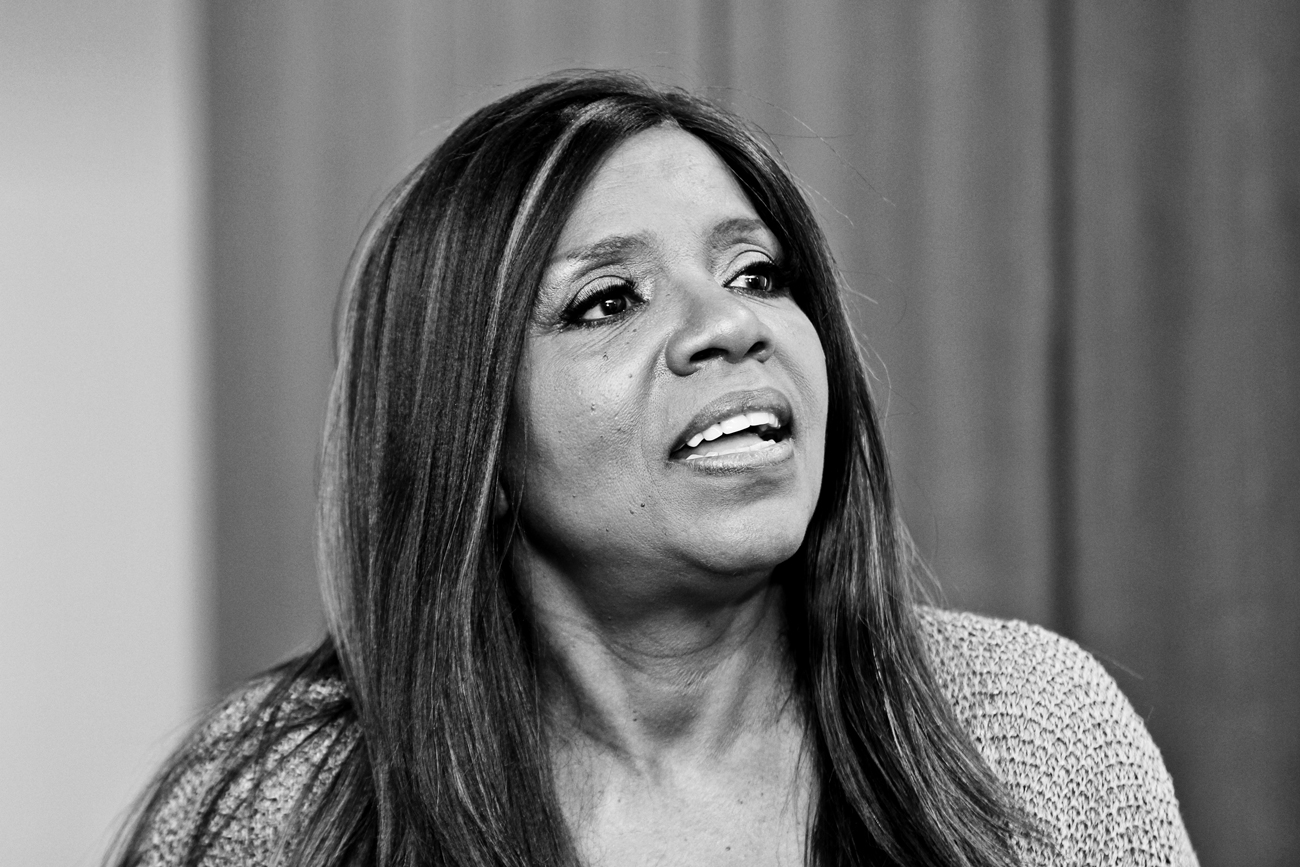This black-and-white photograph features singer Gloria Gaynor. She is wearing a loose-knit sweater which drapes comfortably over her torso. Her long dark hair flows past the frame’s bottom edge and has some light streaks, though the exact details are obscured due to the monochrome nature of the image. Gloria's head is slightly tilted back and upward, angled delicately to the left as she gazes off to the right. Her facial expression suggests she might be in mid-sentence; her mouth is open, revealing both her upper and lower teeth as well as her tongue. She is adorned with what appears to be heavy eyelashes and sparkly eyeshadow, accentuating her expressive eyes even in the grayscale. The backdrop is a mix of light gray tones and features a curtain with visible pleats beside a smooth, texture-less section that resembles a wall.